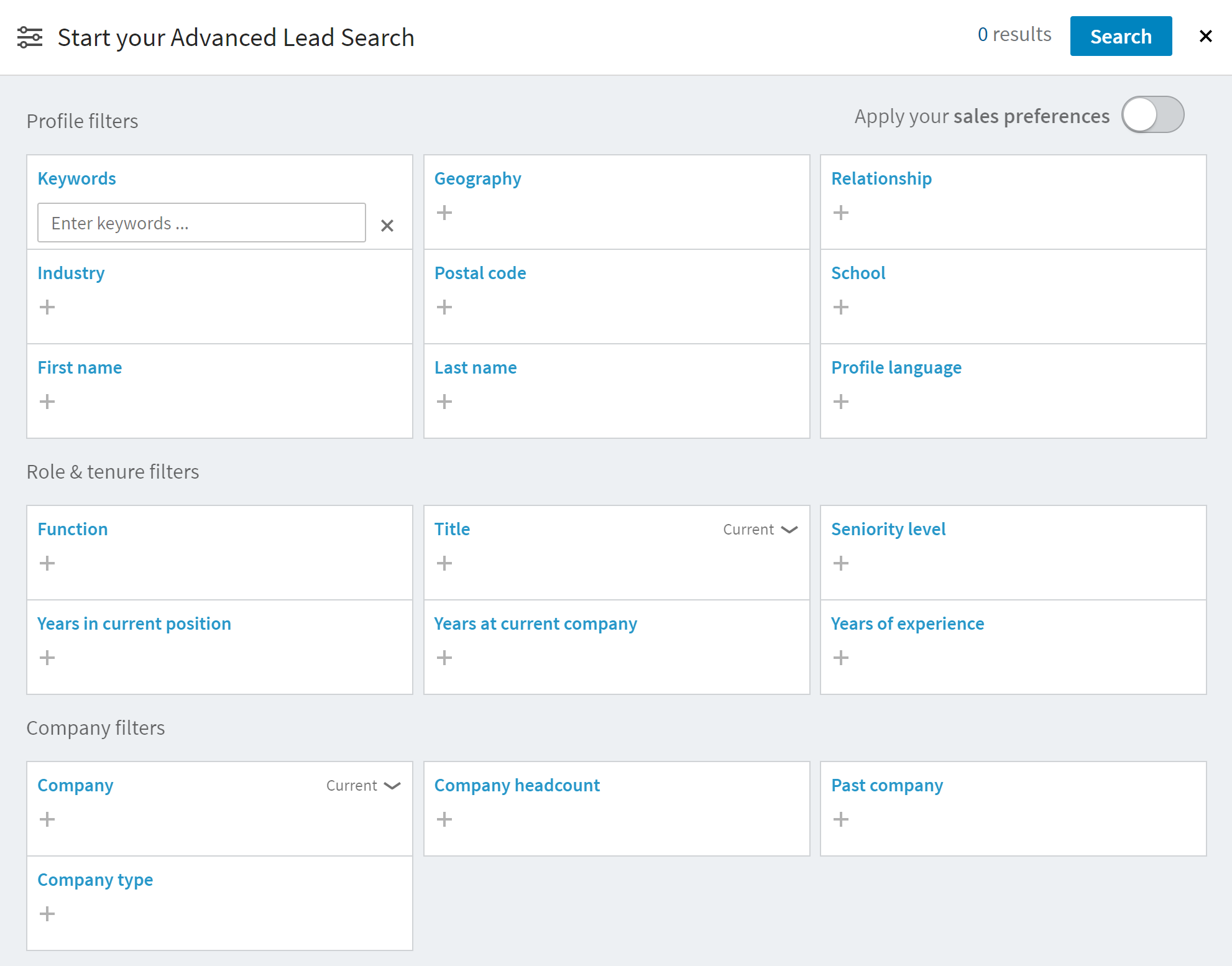The image depicts a user interface for initiating an advanced lead search, primarily aimed at identifying potential clients. The page layout resembles a grid, populated with various editable filters to refine the search criteria. Key filters include "Keywords," "Industry," "First Name," "Last Name," "Geography," and "Postal Code." Additionally, there are more specific subdivisions like "Role," "Tenure," "Function," "Title," "User," and "Company," with further breakdowns under "Company" such as "Company Type" and "Company Headcount." The interface appears capable of searching both individual leads and entire entities. Though detailed information like income or family status might enhance the search, it is presumably more challenging to obtain. The overall purpose of this tool is to provide comprehensive access to varying data points to aid in lead identification.